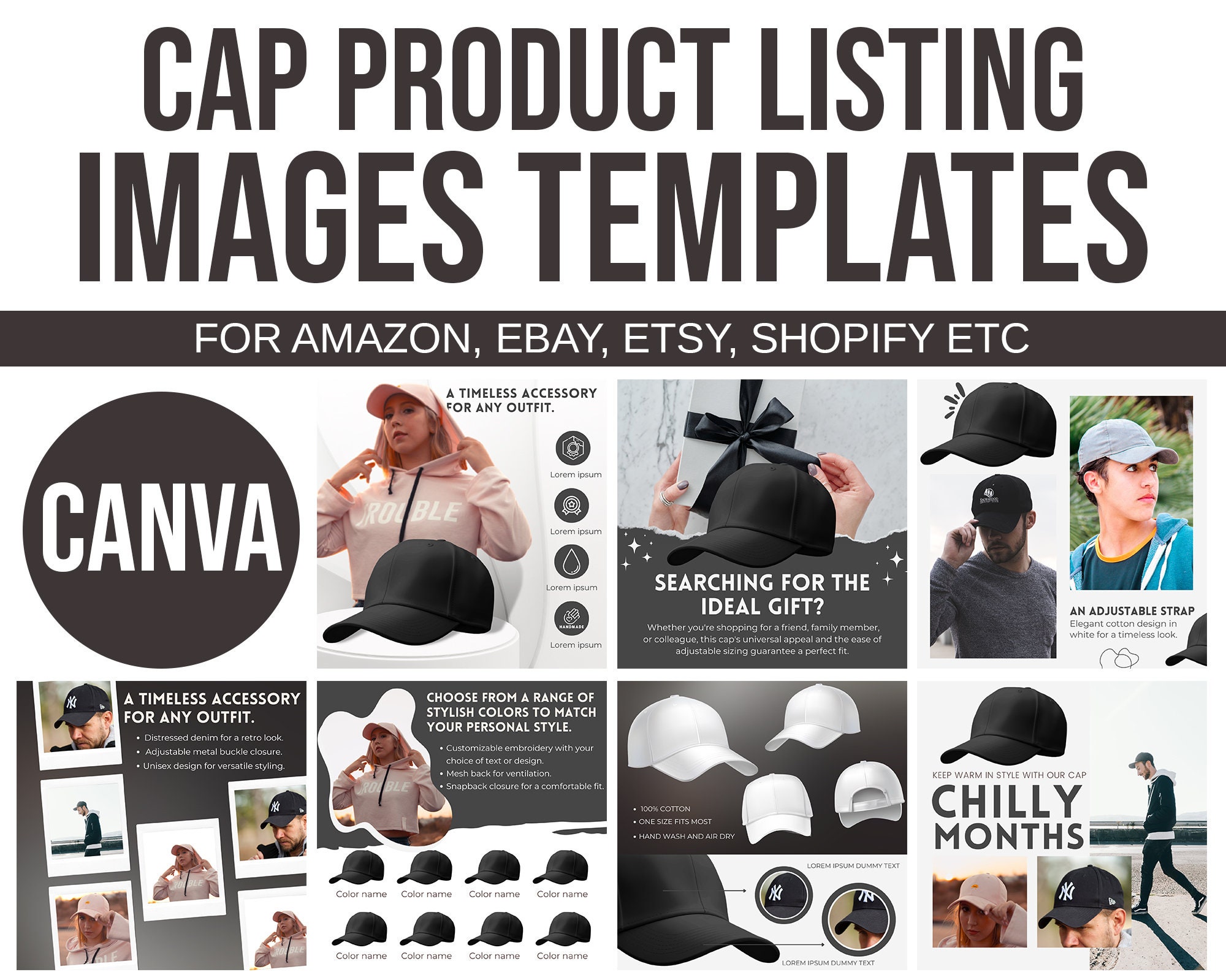This image features a series of meticulously arranged advertising templates for baseball caps, intended for use on online marketplaces such as Amazon, eBay, Etsy, and Shopify. The layout, set against a plain white background without any visible borders, measures approximately six inches wide and four inches high. 

At the very top, two lines of bold dark brown text almost black state "CAP Product Listings, Images, Templates." Directly below this, a quarter-inch-wide dark brown rectangle spans from left to right, containing white text that reads "For Amazon, eBay, Etsy, Shopify, etc."

The central section of the image contains eight distinct sections, each highlighting different aspects of the baseball caps. The first image on the left shows a white background with a dark brown circle and the white text "Canva." To its right, a woman in a pink hoodie and matching cap stands out, captioned "A Timeless Accessory for Any Outfit." Next is a close-up of a black cap labeled "Searching for the Ideal Gift." Following this is another image displaying a man wearing the black cap. Further to the right, another individual is seen sporting a light gray cap, with the text underneath stating "An Adjustable Strap."

Along the bottom, various smaller images are compiled, featuring multiple people showcasing the caps, collectively captioned "A Timeless Accessory for Any Outfit." Continuing to the right, there are two rows of black caps with the caption "Color Name" underneath, and above it, "Choose from a Range of Stylish Colors to Match Your Personal Style." The next segment features a white cap at the top and a black cap below, annotated with "100% cotton, one size fits most, hand wash, air dry." The final image in the corner shows people wearing the caps with the text "Keep Warm in Style with our Cap Chili Months."

Throughout, the caps are showcased in various colors—predominantly black and white—with detailed descriptions emphasizing their versatility, comfort, and style, effectively catering to potential customers on a variety of online platforms.